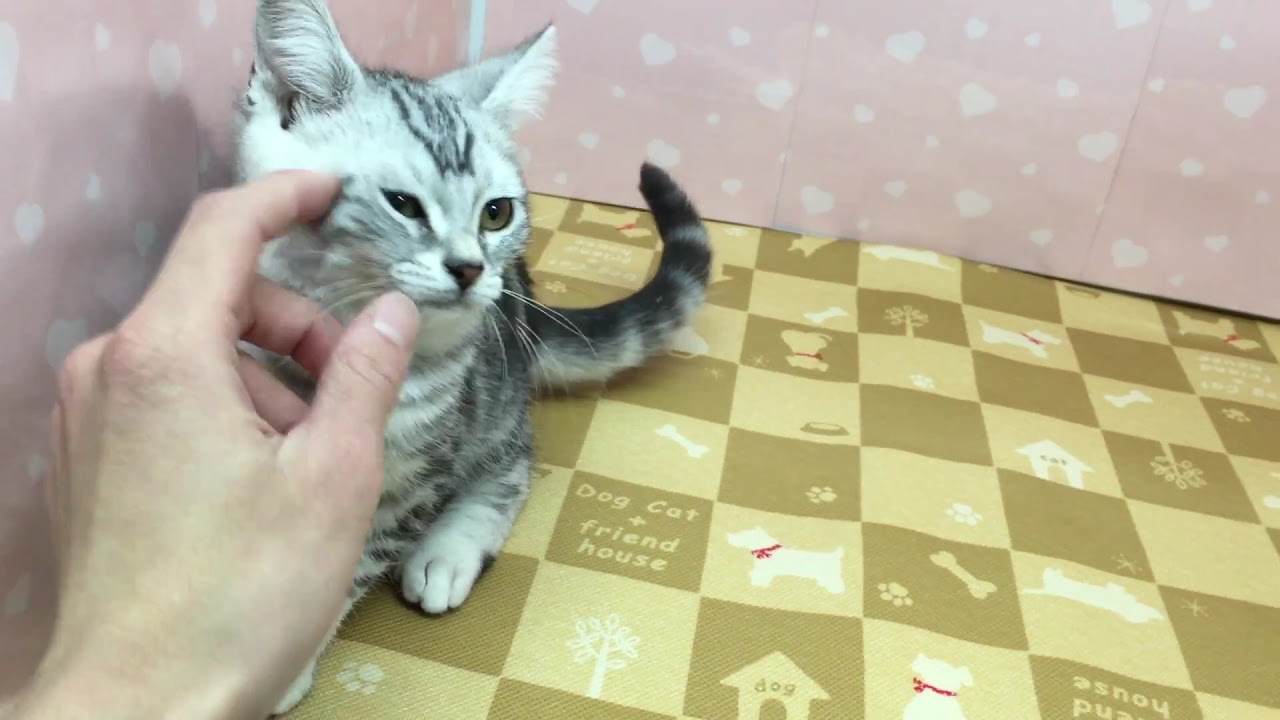In the image, a small black and white kitten with hazel eyes sits slightly off-center to the left, comfortably perched on a cloth with a checkerboard pattern of alternating khaki and light brown squares. Each square contains various pet-themed illustrations, including silhouettes of white dogs, dog bones, dog bowls, paw prints, and a square that reads "Dog, Cat, Plus Friend House" alongside a drawing of trees. The kitten's fur is a mix of black and white with subtle gray streaks, especially around its face, which predominantly features white fur near the whiskers. The kitten's ears are perked up, and its slightly annoyed eyes gaze off to the right. A human hand, extending from the bottom left corner, gently strokes the kitten's cheek, with the thumb aligned near the kitten's mouth and fingers mostly open, touching just below its ears. The kitten's tail extends towards the background. Behind them, the backdrop is a pink wall adorned with white floral or heart patterns, suggesting wallpaper or possibly a decorative paper taped within a cage setting. The scene captures a tender, albeit slightly intrusive, moment between the human and the kitten.